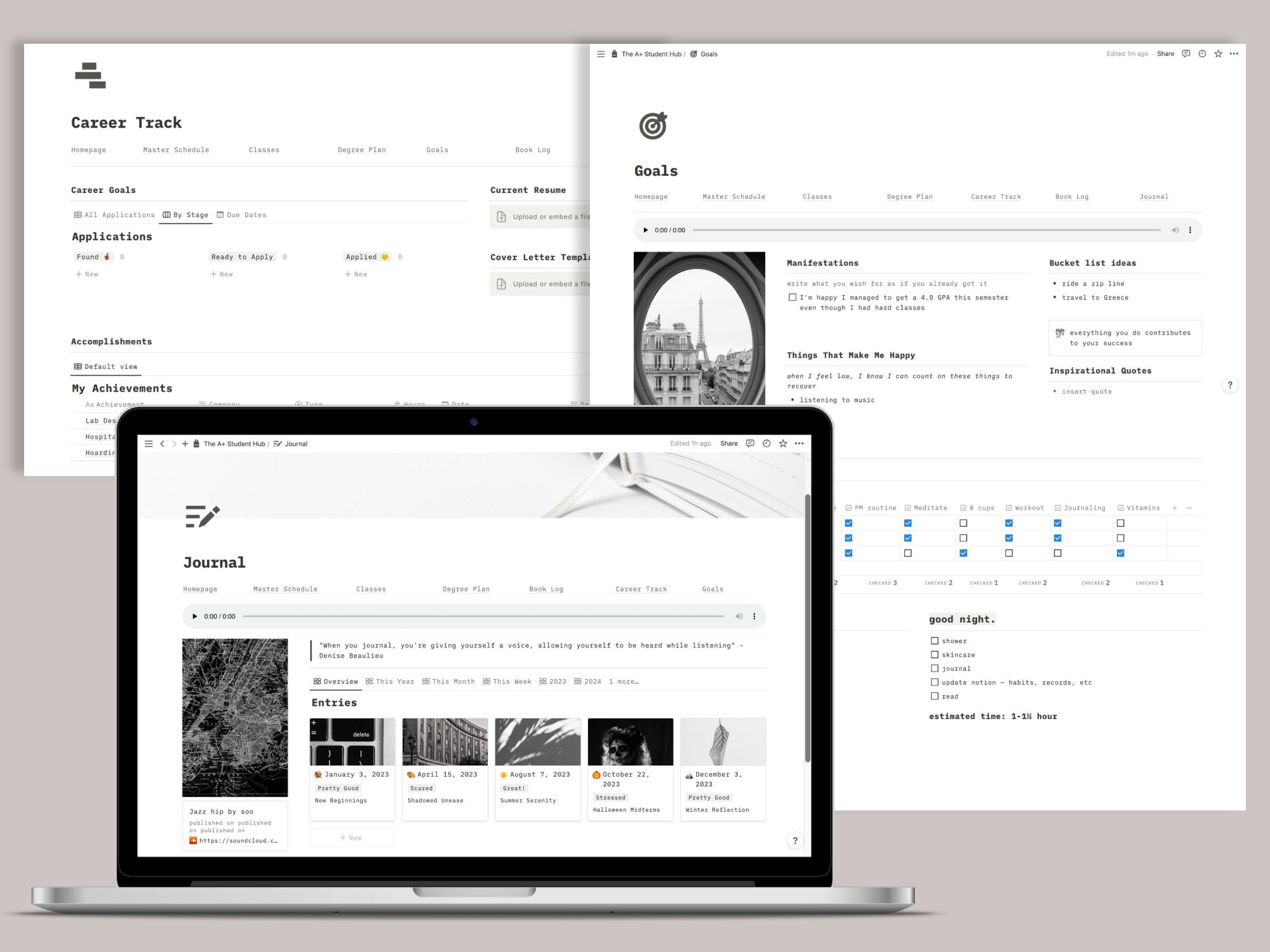This image features a tan-colored background with two prominent, white pop-up portions of webpages and an image of a laptop displaying a webpage. At the top, the white webpage in the background is titled "Career Track" and includes sections labeled Career Goals, Applications, My Achievements, Current Resume, and Cover Letter Template, along with upload spots for these documents. To the right, another similar-looking webpage is visible, titled "Goals," with additional sections labeled Homepage, Master Schedule, Classes, Degree Plan, Career Track, Book Log, and Journal. Below these, there are areas for Manifestations, Bucket List Ideas, Things to Make Me Happy, and Inspirational Quotes.

In the lower portion of the image, a silver laptop with a black border around the screen is visible, displaying a webpage titled "Journal." The screen shows a video ready to be played, titled "Jazz Hip by SOA." A quote on the screen reads, "When you journal, you're giving yourself a voice, allowing yourself to be heard while listening. - Denise Baluya." The setup suggests a workspace dedicated to personal development and career management, combining aspects of goal-setting, self-reflection, and inspiration.